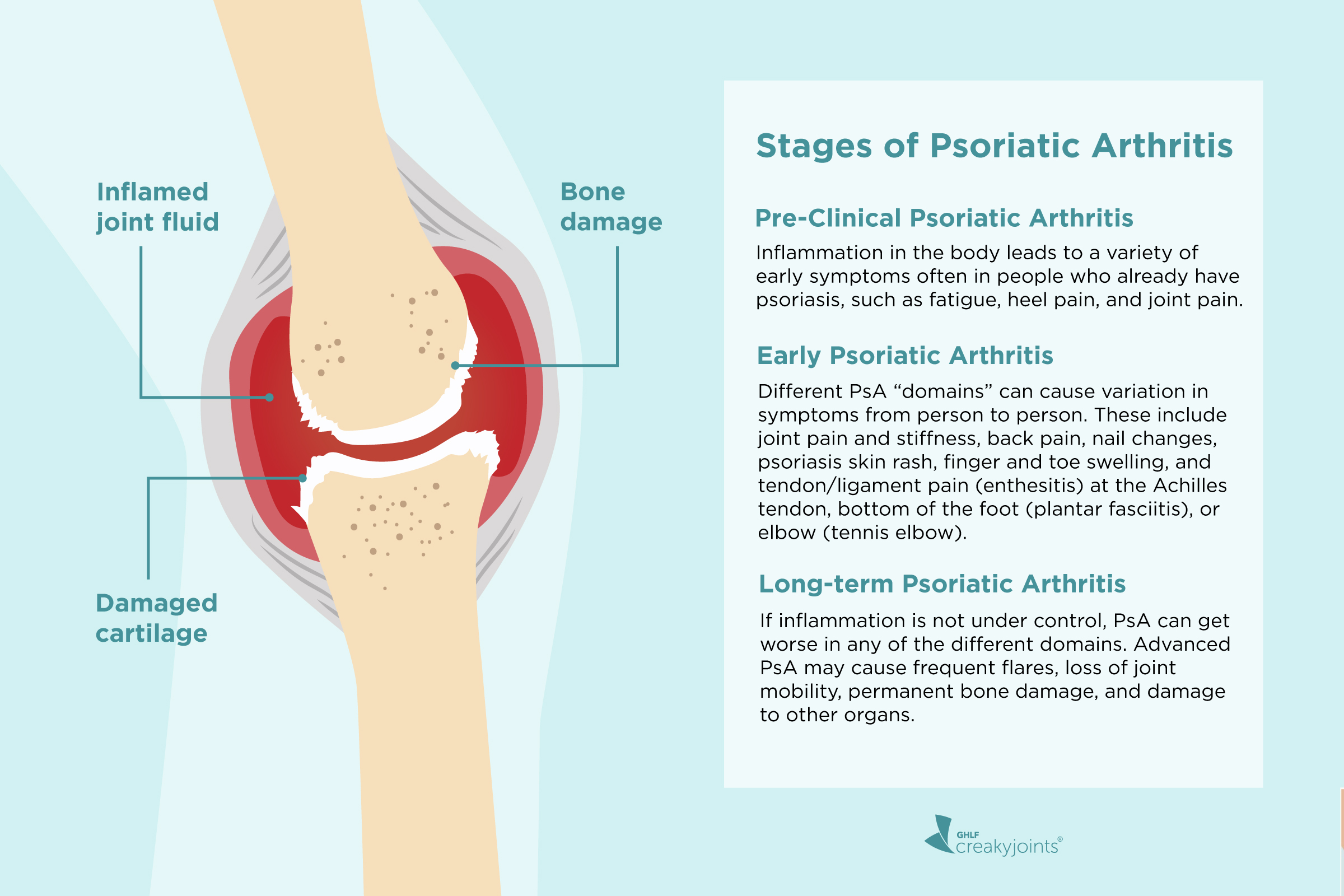This image is a detailed, computer-generated medical diagram illustrating the stages and symptoms of psoriatic arthritis. The diagram, primarily shaded in pale bluish-green hues with tan bones and accents of red and white to indicate inflammation and muscle, serves as an educational tool for patients. On the left side, it features an anatomical depiction of a knee, highlighting bone damage, cartilage degradation, and inflamed joint fluid. The intricate labels and captions point to specific areas, emphasizing the progressive nature of bone destruction and joint inflammation associated with the condition. To the right, there's a structured informational section titled "Stages of Psoriatic Arthritis," which outlines three stages: preclinical, early, and long-term psoriatic arthritis. Each stage is annotated with a smaller, descriptive paragraph in black text, providing insights into the symptoms and progression of the disease. The clear, organized layout and use of color make the information accessible and comprehensible, aiming to inform patients about their condition effectively.